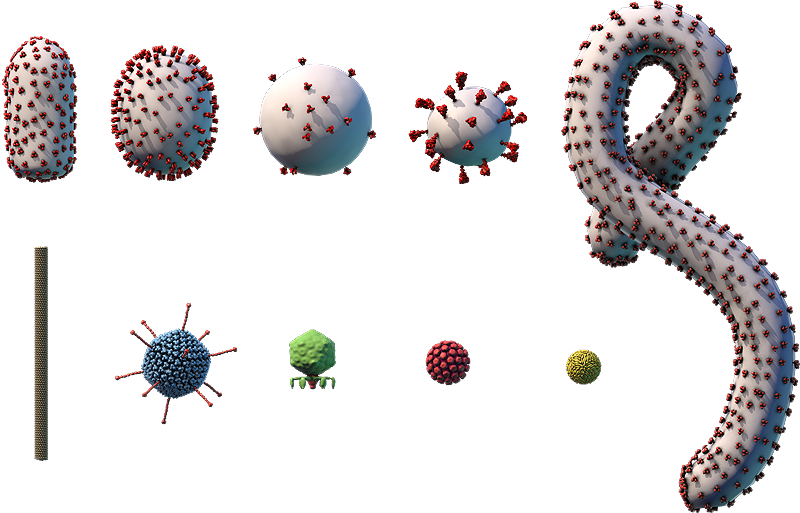The image showcases artistic renderings of various virus-like models arranged against a white background, presented in two rows, each containing four images. The top row includes a series of white shapes with red dots: a cylindrical form, an oblong shape, a large spherical shape, and a smaller spherical shape. The bottom row features more colorful virus models: a spiky blue shape, a small green shape with leg-like extensions, a small red sphere with red spikes, and a small yellowish sphere. Additionally, on the far right of the bottom row, there's a worm-like shape also adorned with red dots. These detailed, computer-animated 3D graphics depict different types of germs or viruses, each showcasing distinct and vivid characteristics.